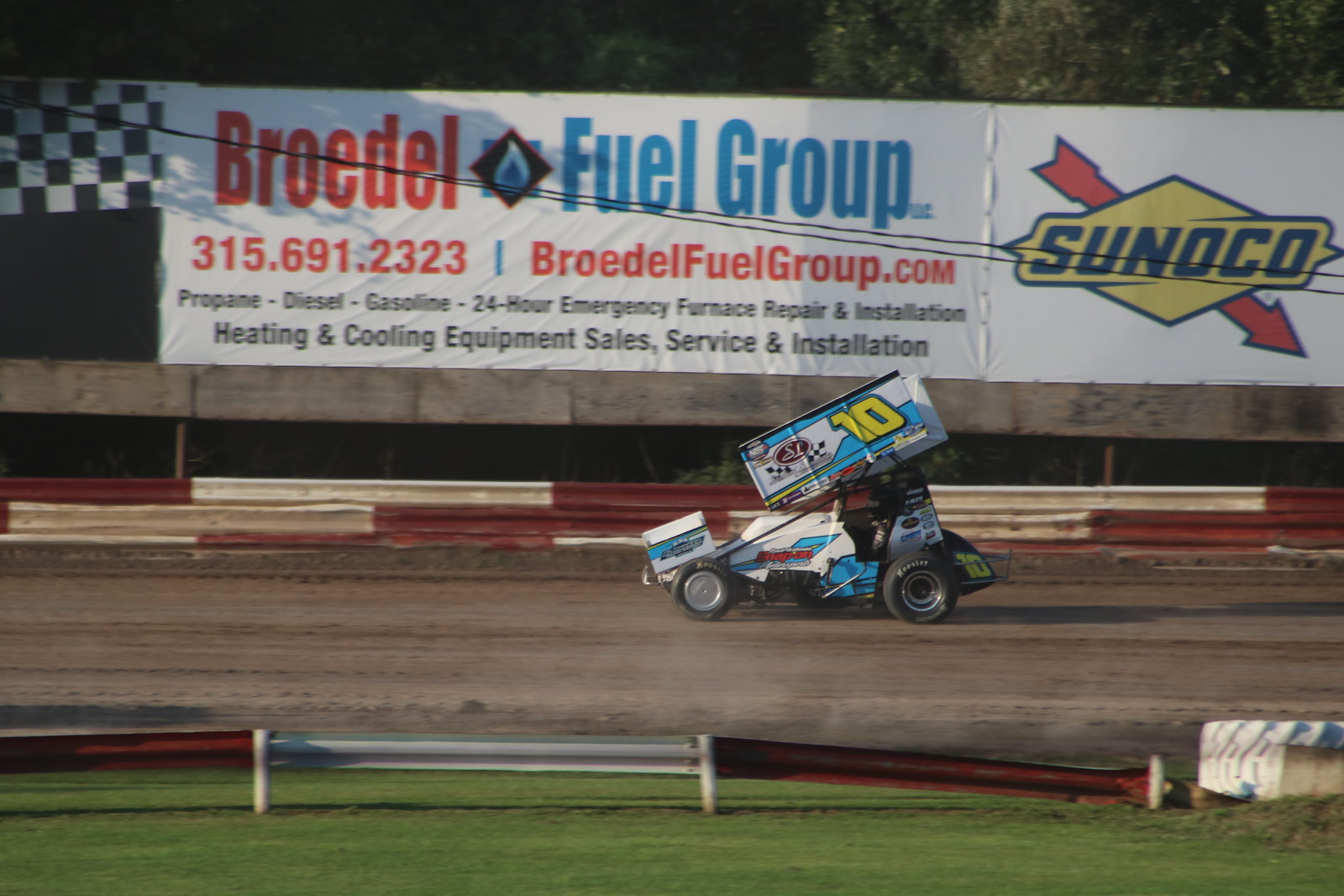This is a photograph of a small race car, resembling a go-kart, on an outdoor racetrack. The car is white with a striking blue number 7 on its side and features a rectangular sign on top displaying a yellow number 10. The car is adorned with various company logos, including a blue square, a blue stripe, a red circle, and a black-and-white checkered flag. The track itself is lined with red and white barricades, and adjacent to the track, there's a grassy area. A prominent white sign along the track reads "Broaddale Fuel Group" and lists their phone number and website. Detailed on the sign are the services they offer: propane, diesel, gasoline, 24-hour emergency furnace repair and installation, as well as heating and cooling equipment sales, service, and installation. Beside this information, the Sunoco logo is displayed in a yellow diamond with a red arrow through it.